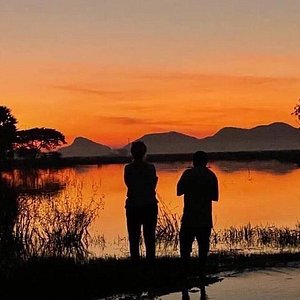The photograph captures the silhouetted figures of two people standing at the edge of a serene lake, their backs to the camera. The scene is set at sunset, with a dusky gray sky illuminated by vibrant hues of orange, peach, and yellow, which beautifully reflect off the calm water. The lake is bordered by a mountain range in the distance, showcasing three distinct peaks in a grayish tone. Surrounding the figures are dark silhouettes of trees and shrubbery, with reeds poking out of the water, creating a textured foreground. The two individuals appear to have their arms in front of them, suggesting they might be carrying something, potentially hinting at a fishing trip. The image is meticulously composed, possibly taken by a professional, capturing the tranquil and contemplative atmosphere of the moment without any text or additional distractions.